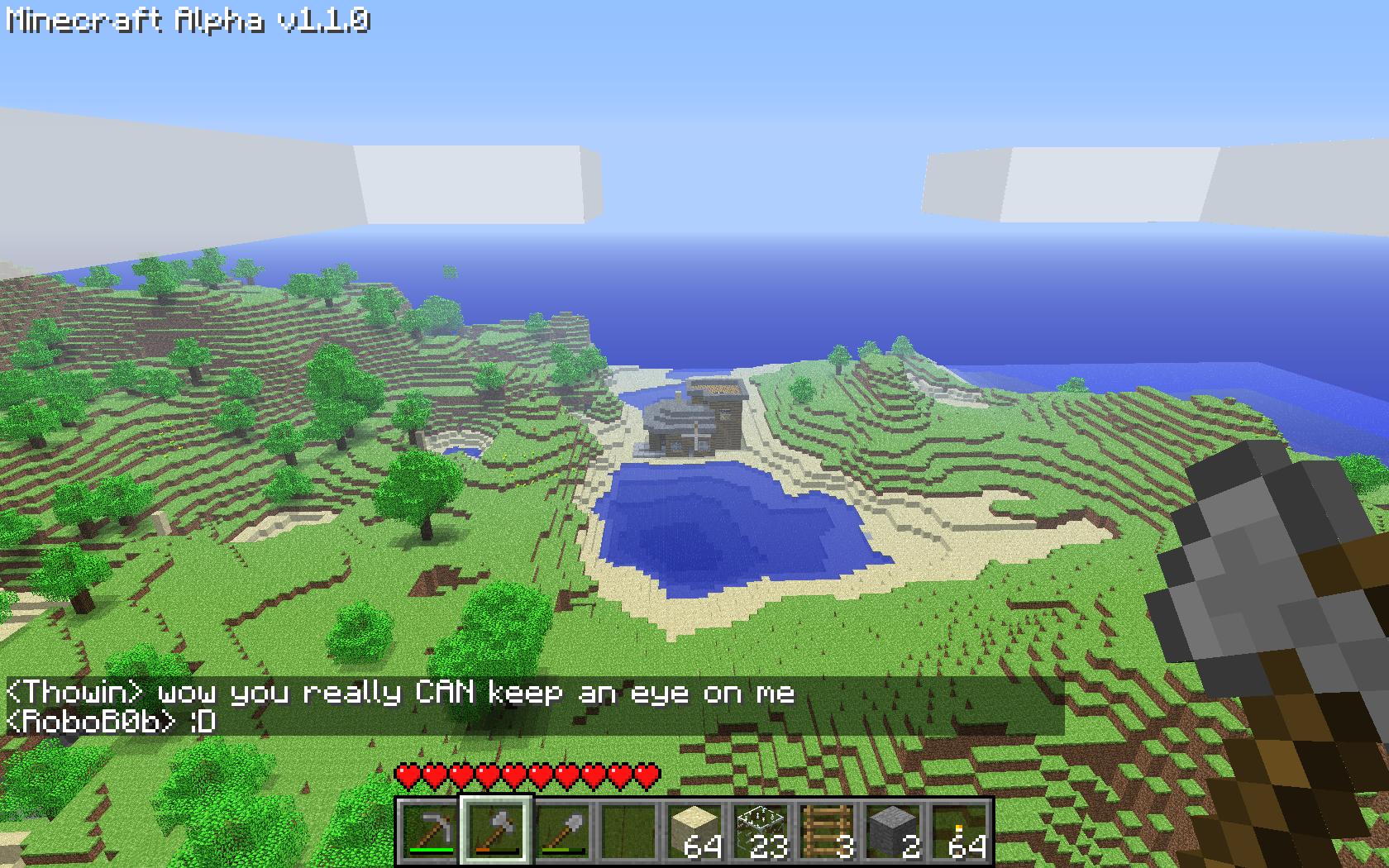The image is a screen capture from the Minecraft Alpha v1.1.0 video game, as indicated in white text in the upper-left corner against a light blue sky. The landscape features a distinctly retro and blocky aesthetic, reminiscent of Roblox, with lush green hills and mountains. In the center, there is a small pond encircled by sand, beside a two-story gray structure with varying roof heights. The background showcases a dark blue ocean seamlessly transitioning into the sky.

In the foreground, an overlay text window displays an in-game conversation: "Tawan says, 'Wow, you really CAN keep an eye on me'"—with 'CAN' capitalized. "RoboAOB" responds with a smiley face emoticon ":D". Just below this text, a series of red hearts signify the player's remaining lives, accompanied by various icons representing their inventory of materials and tools. Additional elements include gray and white block structures on both sides of the image, integrated into the green landscape.